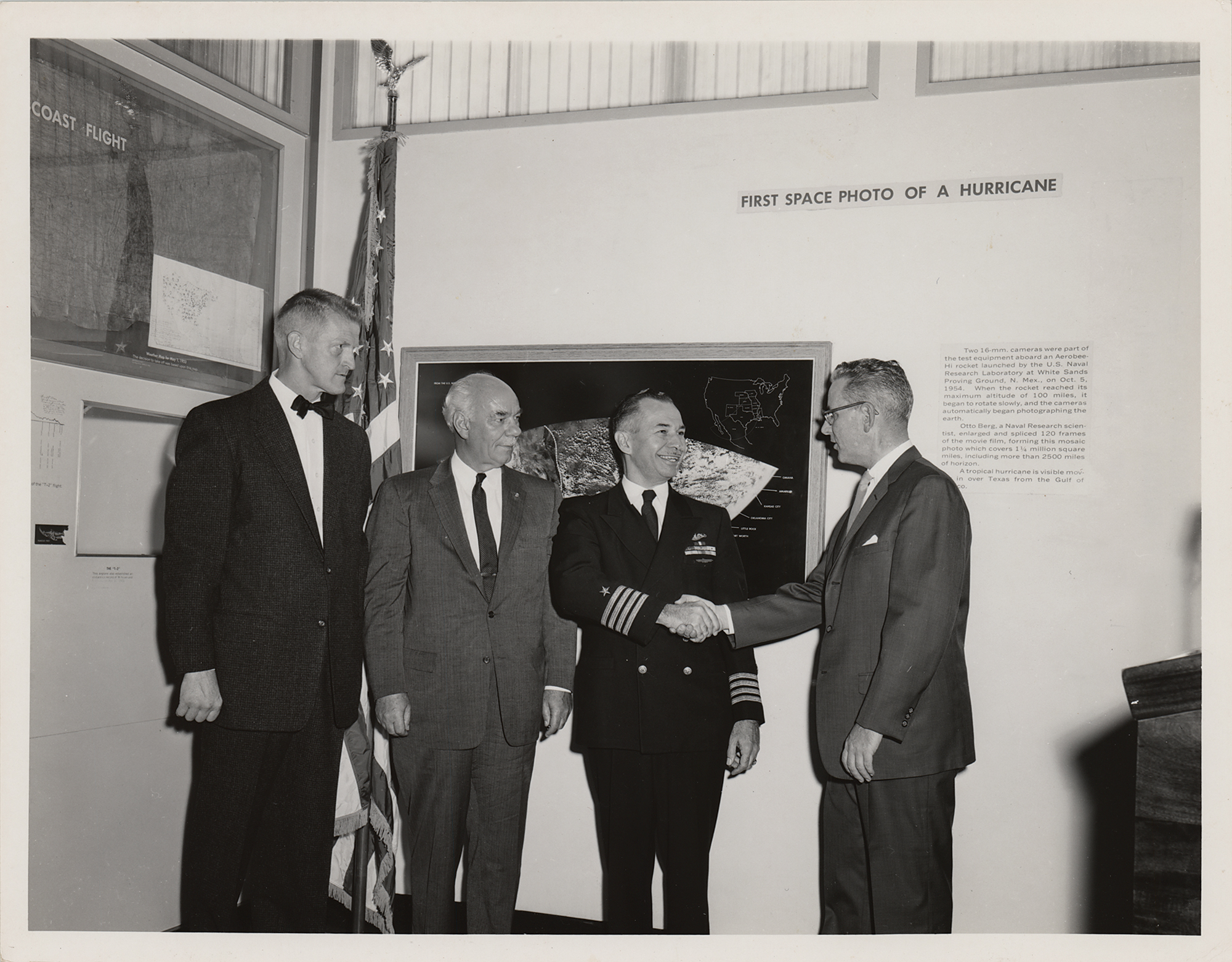This is a detailed black-and-white photograph depicting an important historical moment. The backdrop of the image is a white wall featuring prominently the text "First Space Photo of a Hurricane" in black letters. Beneath this header is a detailed description outlining how two 16mm cameras were part of the test equipment aboard an Aerobee high rocket launched by the U.S. Naval Research Laboratory at White Sands Proving Ground NMAX on October 5th, 1954. The inscription explains that as the rocket reached its maximum altitude of 100 miles, it began to rotate slowly, enabling the cameras to automatically capture photographs of the Earth. However, part of this text is grainy and hard to read.

In the center of the image are four men, all dressed in suits, standing in front of this wall. To the left, a tall man in a black suit and bow tie stands beside an older, balding man with white hair wearing a dark suit and tie. To their right, a man in a military uniform adorned with four stripes and stars on his sleeves can be seen shaking hands with another man who has black-framed glasses and a dark grey suit, complete with a white pocket square and a grey tie. There is also an American flag, crowned with an eagle, on a black pole behind them, adding a patriotic element to the scene. In the background, partially obscured by the men, appears to be a large framed photograph, perhaps the historic space photo of the hurricane, accompanied by additional text that is too small to decipher. The overall setting suggests a formal and significant occasion, commemorated by this gathering of distinguished individuals.